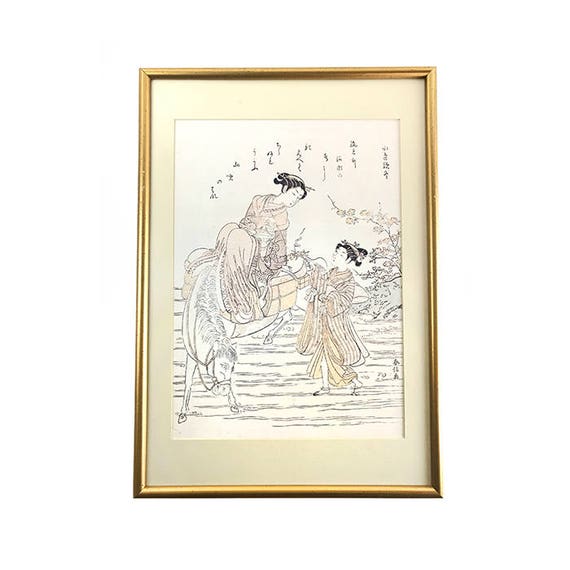This image features a framed painting with a golden (or brass) wood frame and a cream-colored mat, set on a light beige background. The central scene depicts two Asian figures, likely from ancient Japanese or Chinese times, based on the traditional attire and hairstyles. The older figure, dressed in a kimono robe, is riding a small horse or donkey laden with luggage, and is seen leaning toward the center of the image. She appears to be engaged in conversation with a young girl standing on the ground beside her, also wearing a kimono robe. The backdrop includes a white sky with Asian script above them, adding to the cultural context, and a grassy field with trees and plants nearby. The artwork is rendered in black and white, emphasizing the detailed interaction between the two figures amidst a serene outdoor setting.